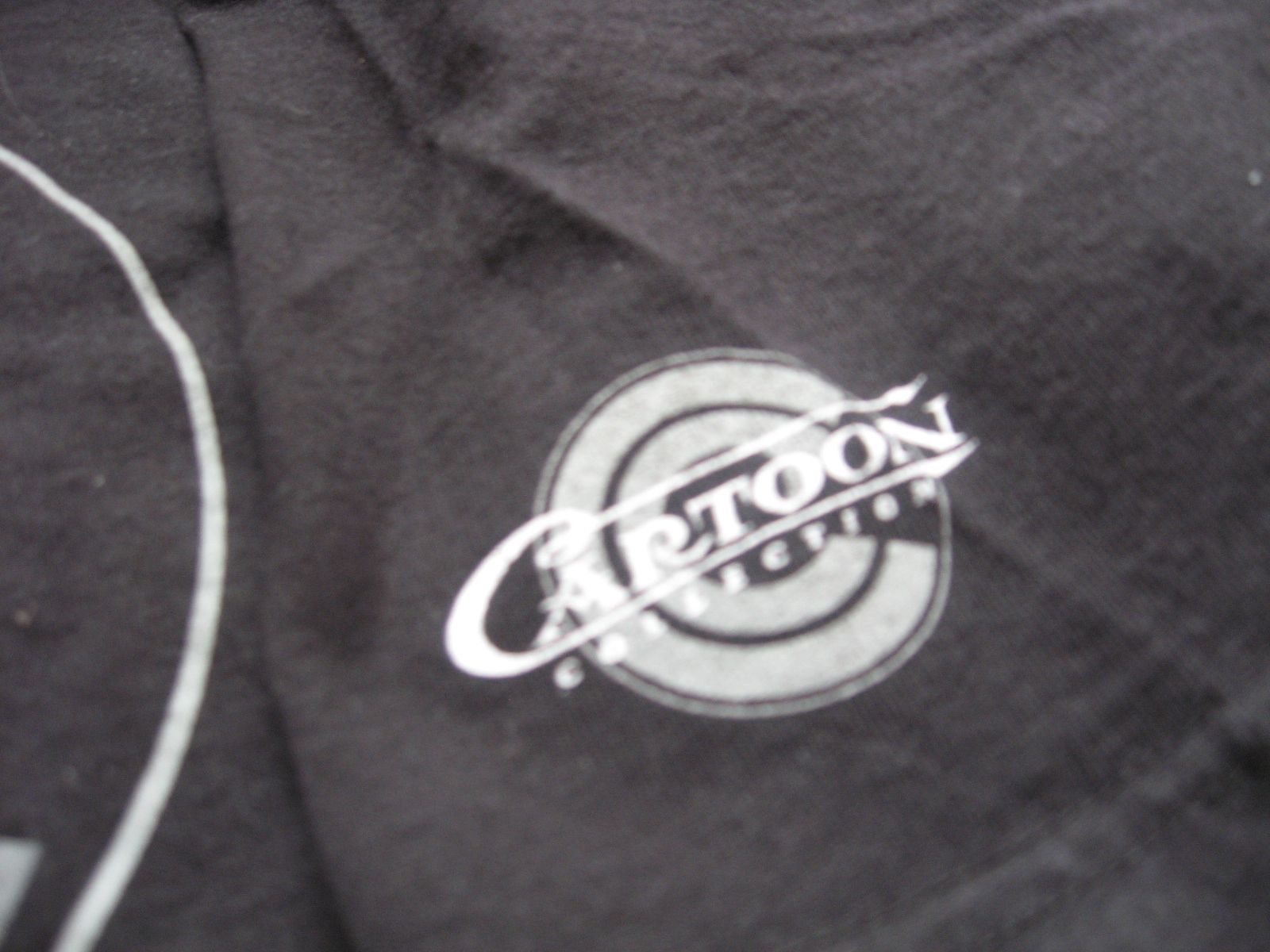This detailed black-and-white close-up photograph captures the texture and intricate details of a fabric item, likely a piece of clothing. The fabric has a distinct texture with visible creases that give it a tactile feel. At the center of the image, a prominent logo insignia features a circular design. Within this circle, there is a stylized letter "C" composed of two thick stripes. Overlaying this insignia is the word "Cartoon" in large, elegant script letters, with the smaller word "Collection" printed below in very fine, white ink. Additionally, on the left side of the image, there is a partially visible white semi-circle, suggesting another element of the design that is cut off at the edge of the photograph. The interplay of the fabric's texture with the bold and subtle elements of the logo creates a visually compelling composition.